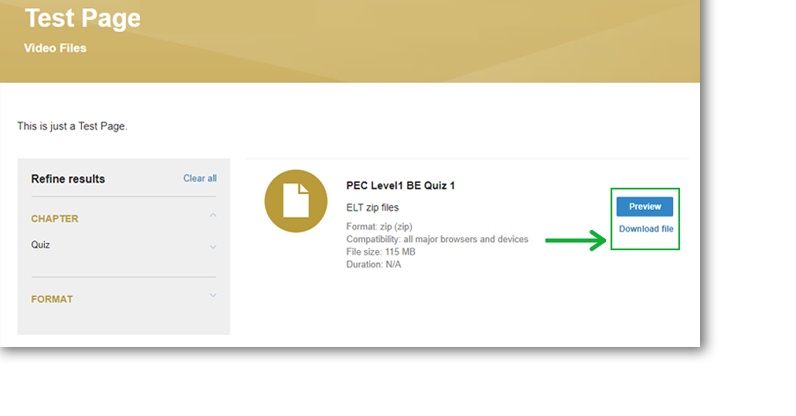This image depicts a test page, prominently featuring a large golden banner at the top with the text "TEST PAGE" in bold white letters. Below this banner, it says "Video Files" in smaller font. 

On the left-hand side of the page, a sidebar includes the text "This is just a test page." Beneath this, there's a small grey menu box that reads "Refine Results" with a "Clear All" option next to it. 

Further down the sidebar, the word "Chapter" appears in golden font, followed by "Quiz" beneath it. Below "Quiz," "Format" is also written in golden font and is accompanied by a small image icon of a PDF document which reads "BEC Level 1 BE Quiz 1."

Continuing downward, the text reads "Elt zip files, format zip compatibility, all major browsers and devices." Adjacent to this text is a large horizontal green arrow pointing towards a box with a green outline containing the text "Preview Download File." 

Below this box, additional text states "File size: 115 MB" and "Duration: Not Available."